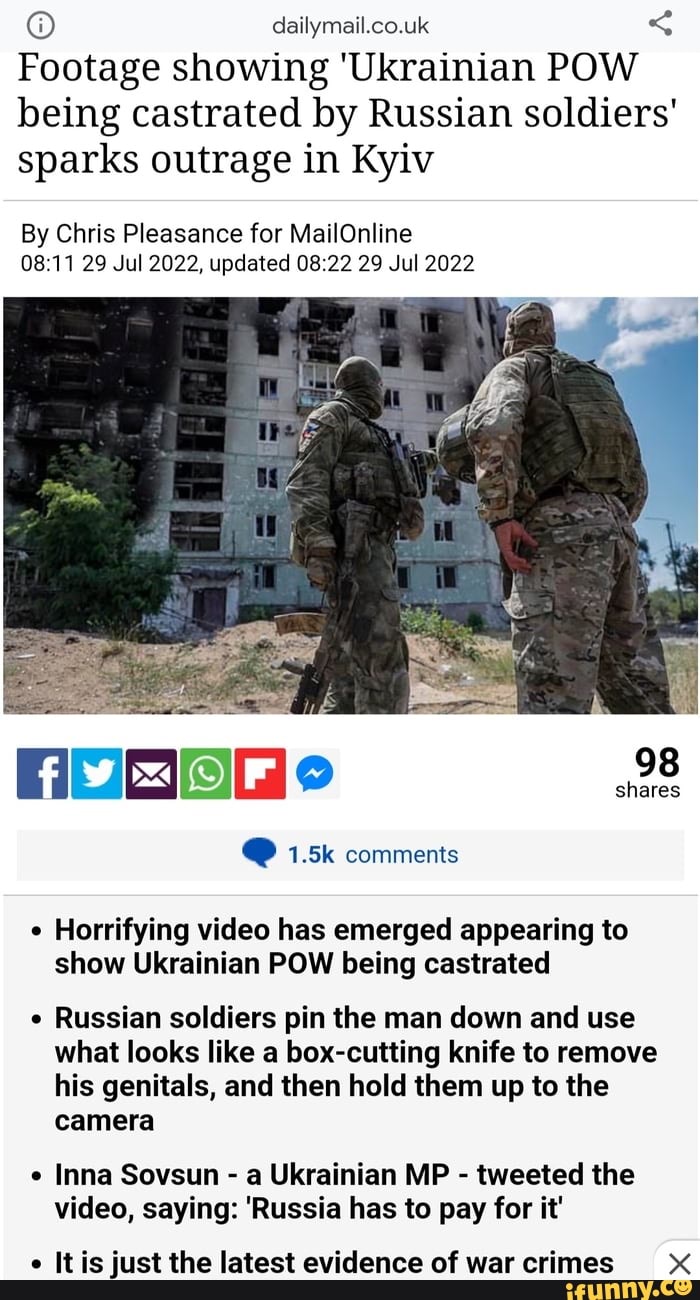The image is a screenshot from a mobile device, displaying a narrow vertical rectangle typical of such captures. At the top of the screenshot, a gray bar contains a web address reading "dailymail.co.uk," indicating it's from a news website. The prominent headline reads, "Footage showing Ukrainian POW being castrated by Russian soldiers sparks outrage in Kiev," credited to Chris Pleasence for Mail Online. The article was first published at 8:11 AM on July 29, 2022, and was last updated at 8:22 AM the same day.

Beneath the headline, a large rectangular photograph depicts a bombed-out building in the background, with bushes and trees visible to the left side and dirt covering the ground. In the foreground, on the right side, stand two soldiers dressed in green camouflage attire with hoods and masks obscuring their faces. Their hands, however, are visible and reveal them to be Caucasian.

At the bottom right of the image, a label shows it has "98 shares" and "1.5k comments." Below the photograph, a gray text box contains the following black text: "Horrifying video has emerged appearing to show Ukrainian POW being castrated. Russian soldiers pin the man down and use what looks like a box cutting knife to remove his genitals and then hold them up to the camera." There is additional text under this description, highlighting the gruesome and disturbing nature of the content.